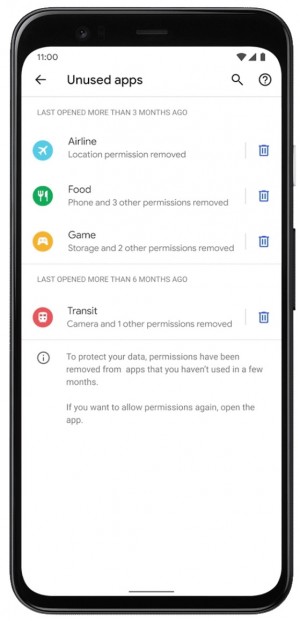**Detailed Caption:**

This image is a detailed mock-up of a smartphone screen showcasing a page dedicated to unused apps, likely intended as a part of an educational guide on managing smartphone applications. The outer bezel of the smartphone is gray, while the inner bezel is black. At the top left corner of the screen, the time is displayed as '11', without an AM or PM indicator, suggesting the use of military time.

On the top right corner, there are icons indicating a full Wi-Fi signal, a full cellular signal, and a battery indicator.

On the left side, slightly below the top edge, there is a black arrow pointing to the left, accompanied by bold black text that says "Unused Apps." On the right side, there is a bold black magnifying glass icon and a bold black circle with a question mark inside it. Below these elements, a thin gray line spans the width of the screen.

Under this line, a message in all capital letters reads "LAST OPENED MORE THAN THREE MONTHS AGO." 

The section beneath this message includes:
1. A cyan blue circle with a white silhouette of an airplane labeled "Airplane" in bold black text, and beneath it, gray text that reads "Location permission removed."
2. A green circle featuring a white fork and knife icon, labeled "Food" in bold black text, with gray text below saying "Phone and three other permissions removed."
3. An orange circle with a white game controller icon, labeled "Game" in bold black text, and underneath, gray text stating "Storage and two other permissions removed."

Separated by two thin gray dotted lines, another message reads "LAST OPENED MORE THAN SIX MONTHS AGO."

This section features:
1. A red circle with a white bus icon, labeled "Travel" in bold black text, with gray text underneath indicating "Camera and one other permission removed."

The last section shows a black circle with a black eye icon. Next to it, a message in black text reads: "To protect your data, permissions have been removed from apps that you haven't used in a few months. If you want to add permissions back, open the app."

Each app icon in the list has a blue trash can icon next to it, indicating the option to delete these unused apps.